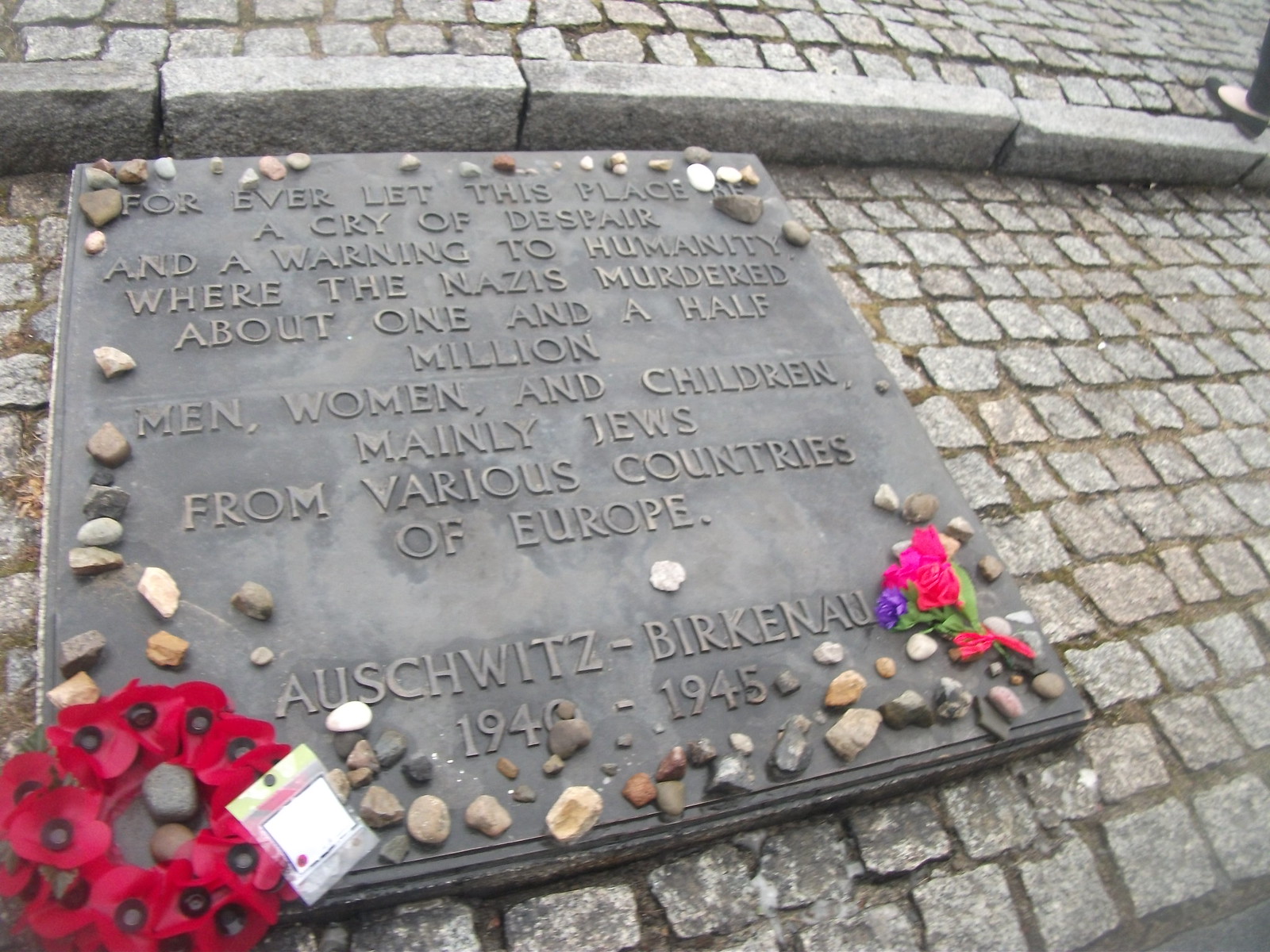The image is a landscape-oriented color photograph of a memorial plaque affixed to a rock wall surface. The plaque is composed of gray squares held together by brown-colored grout. It bears an inscription that reads, "Forever let this place be a cry of despair and a warning to humanity where the Nazis murdered about one and a half million men, women, and children, mainly Jews, from various countries of Europe. Auschwitz-Birkenau, 1940-1945." Surrounding the plaque are numerous pebbles and flowers. Specifically, in the bottom left corner, a ring of red flowers, possibly poppies, can be seen, with a clear plastic bag attached to it. Additionally, there are some pink and purple flowers in the bottom right corner. A person’s leg, dressed in black pants and a black shoe, steps up visible in the upper right corner, revealing their white skin. The setting evokes a somber, reflective mood, capturing the essence of photographic representational realism.